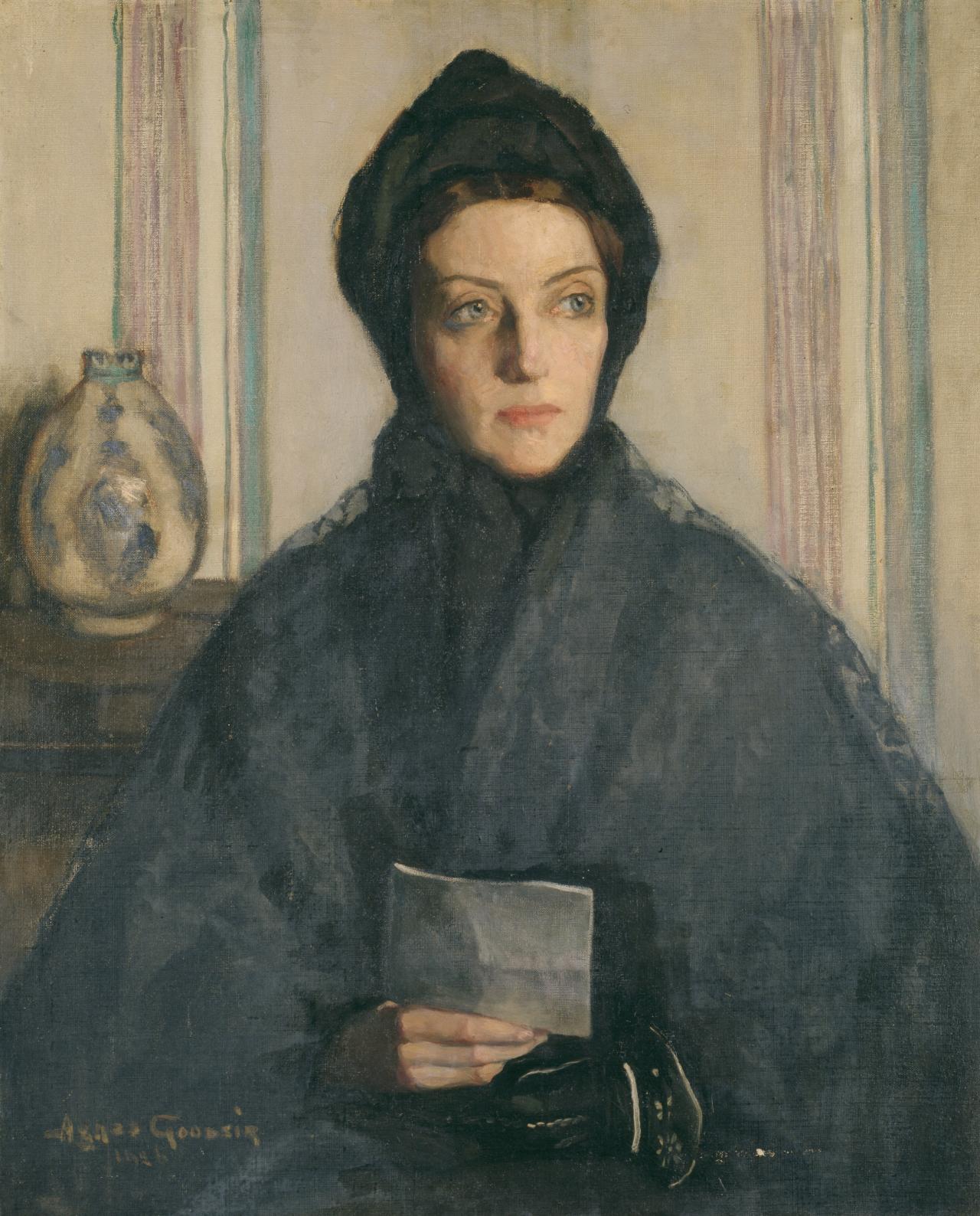This detailed painting portrays a serene-looking woman with a fair complexion, blue eyes, and pink lips. She has slightly rosy cheeks and brown hair parted down the middle, partially visible beneath a black bonnet. She wears a black robe with a lace shawl draped over her. Her eyebrows are slightly raised as she gazes to her left. Her right hand, which is ungloved, holds a white piece of paper, while her left hand, clad in a black glove featuring a detailed design on the cuff, rests at her side.

Behind her, the setting includes a wooden cabinet adorned with a blue and white vase. The backdrop is a cream-colored wallpaper with vertical stripes of blue, white, pink, and purple. In the lower left corner of the painting, the artist's name can be seen, possibly reading "Agnes Gooding," though the signature is partially legible. The artist has deftly captured a lifelike and tranquil representation of the woman, making the painting almost photographic in its realism.